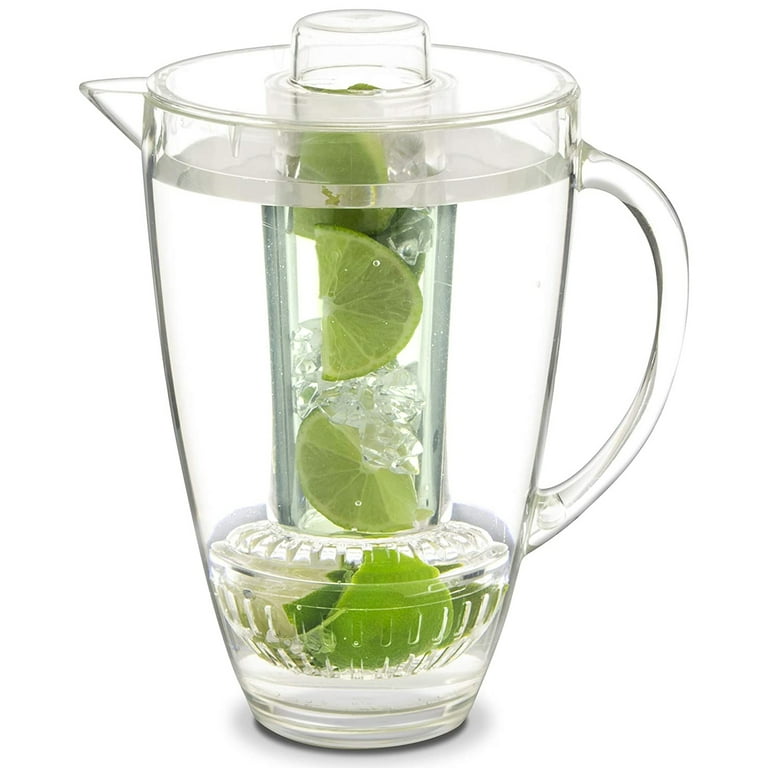The image depicts a clear infusion pitcher, likely made of plastic or possibly acrylic, designed for infusing flavors into liquids. The pitcher stands upright with a modern design that tapers from a wider top to a narrower bottom. It features a flat, easily removable lid with a handle on top and a V-shaped spout positioned on the left. The right-hand side is equipped with a handle, possibly plastic or glass. Inside the pitcher, a center tube extends through the length of the body, terminating into a cylindrical compartment at the bottom. This compartment includes holes that allow the properties of its contents—ice and lime wedges, visible inside the tube—to infuse into the surrounding liquid, which is clear, likely water. The pitcher appears to be filled about a quarter of the way with water.